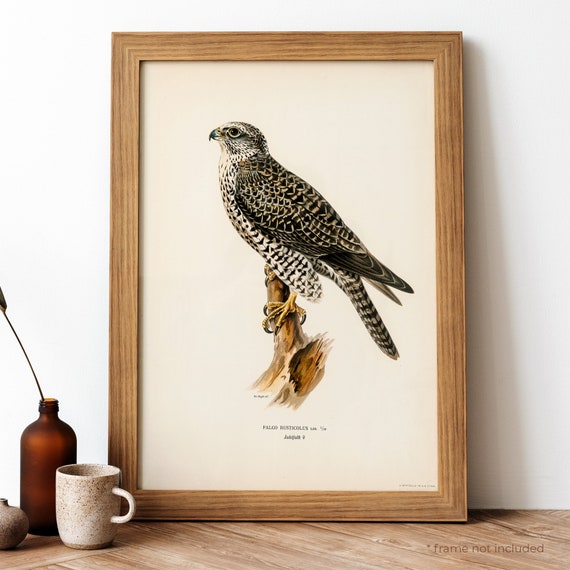In this staged photograph of an ink drawing, a finely detailed illustration of a hawk or falcon-like bird is prominently featured. The bird, which sports speckled black, brown, and white feathers along with a large eye and small beak, is perched on a branch. The drawing is framed in a light oak-colored frame and rests against a white wall with light wood-grain flooring that matches the frame's hue. Accompanying the framed drawing are a white speckled coffee mug and a copper-colored apothecary bottle with a single floral stem, adding a homely touch to the scene. The drawing, centered against a white background, includes some text, likely labeling the bird, although it is too blurry to read. The overall aesthetic features a palette of black, white, beige, and brown.